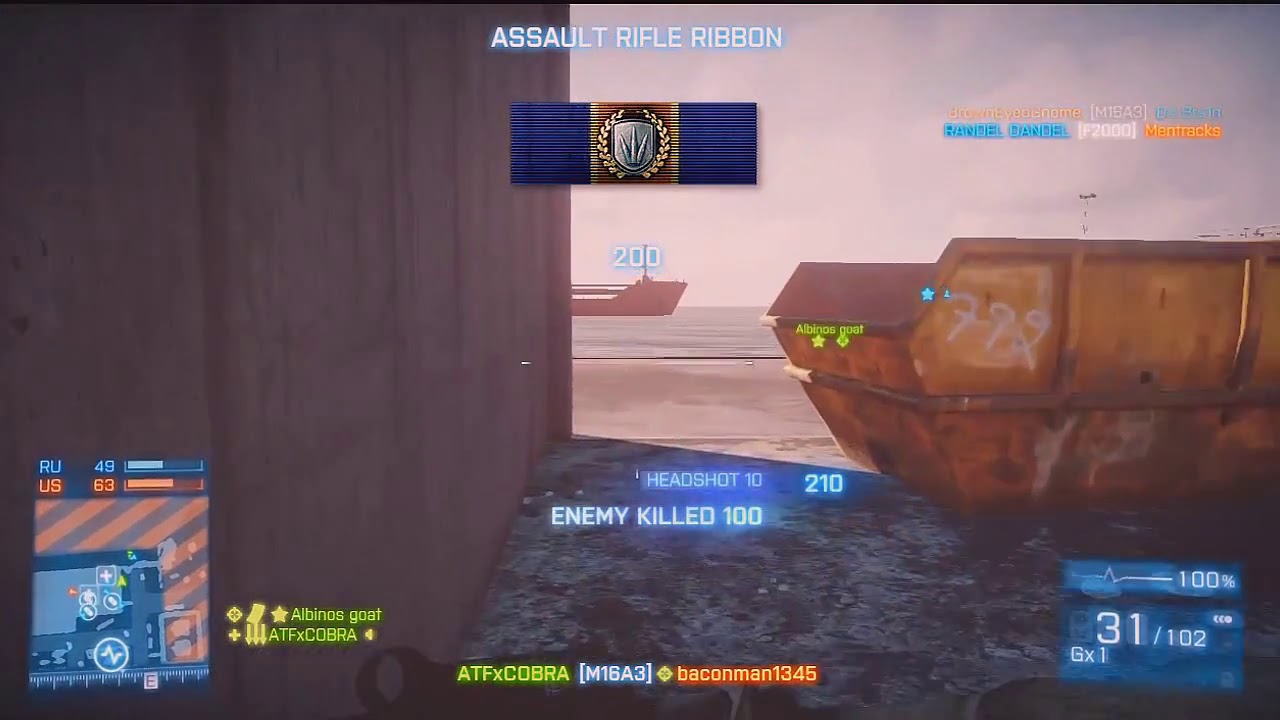This detailed caption synthesizes the inputs into a single cohesive description:

This screenshot from the video game Battlefield showcases a first-person shooter scene set at a ship dock by the ocean. Dominating the foreground is a rusted container adorned with graffiti, positioned centrally. To the right of the screen, there's an orange dumpster, while a gray cement wall occupies the left. The background features expansive water and a large container ship sailing by. Atop the screen, there's an "Assault Rifle Ribbon" icon, displaying a medal with blue, silver, and brown hues. Just below this, the on-screen text details achievements: "Headshot 10, Enemy Killed 100", visibly highlighted in a LED-like blue light. The lower left corner reveals a mini-map indicating a match between Russia and the US, with the scoreboard showing RU49US63. Additionally, vital player information such as health and ammo is displayed on the bottom right, with the username 'ATFX Cobra' prominently featured.